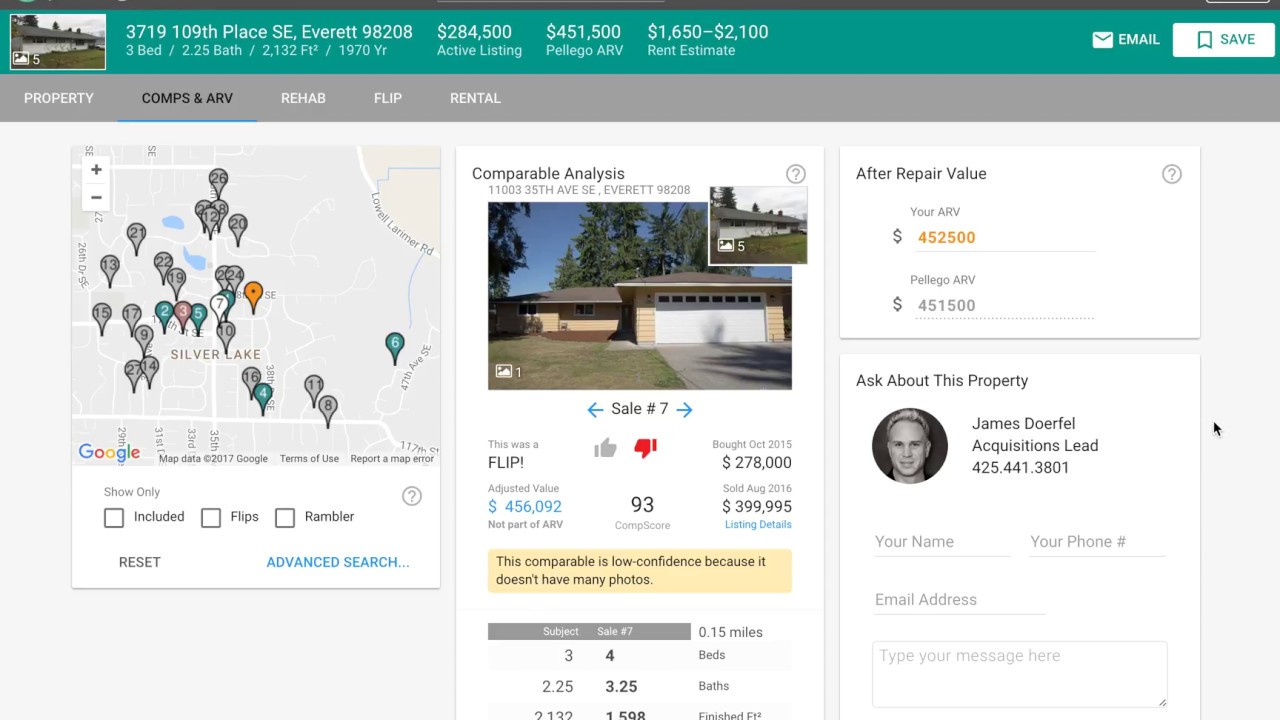This is a screenshot of a real estate website. At the top of the page is a green bar. On the left side of this bar, there is a thumbnail image of a house. Next to the thumbnail, the address of the property is listed as "3719 109th Place Southeast, Route 98208." Below the address in white text, additional property details are provided: "3 bed / 2.25 bath / 2132 sq. ft. / Built in 1970." The listing price is indicated as "$284,500 Active Listing," and the After Repair Value (ARV) is stated as "$451,500 Pelego ARV." A rent estimate ranges from "$1,650 to $2,100." On the right side of the green bar, there are two buttons: "Email" and "Save." The "Save" button has a white background with green text, while the "Email" button is white. Below the green bar is a grey bar featuring five buttons labeled: "Property," "Comps and ARV," "Rehab," "Flip," and "Rental."